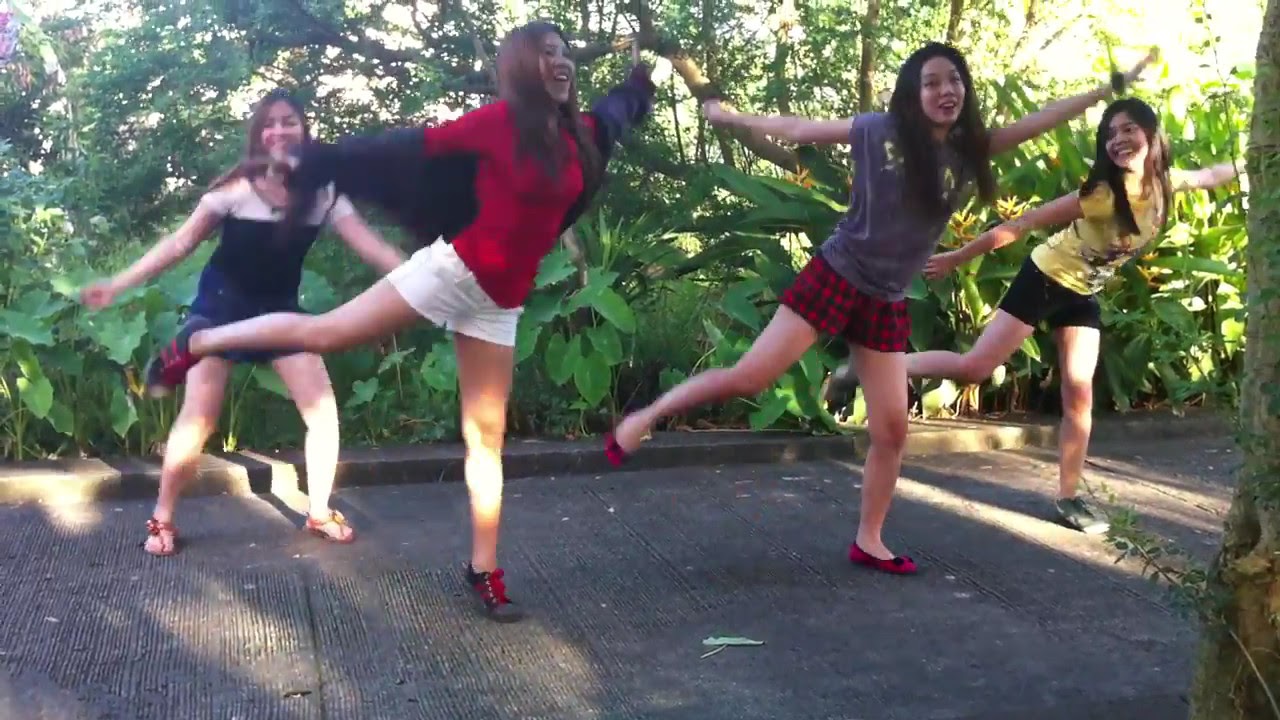In this photograph, four girls are captured performing a coordinated dance routine outdoors in front of lush, tropical plants with oversized leaves. The background foliage appears almost like a botanical garden, adding a vibrant, green backdrop to the scene. The ground they are dancing on has a green, possibly artificial, surface resembling a sidewalk. All four girls are smiling brightly and looking directly at the camera, radiating joy and excitement.

From left to right, the girls are dressed in distinctive outfits: the leftmost girl is wearing a white and blue shirt with blue shorts, the next girl to her right is in a red long-sleeved shirt paired with white shorts. The third girl is dressed in a grey short-sleeved shirt and red and black plaid shorts, while the rightmost girl sports a yellow short-sleeved shirt with black shorts. Three of them have one leg raised and are balancing on the other, synchronizing their movements with arms outstretched as if trying to take flight. Meanwhile, the leftmost girl appears slightly out of sync, with both her legs planted on the ground but raising her arms in an effort to match the pose. Each girl has long, dark hair cascading below their shoulders, enhancing the dynamic and lively atmosphere of the photograph.